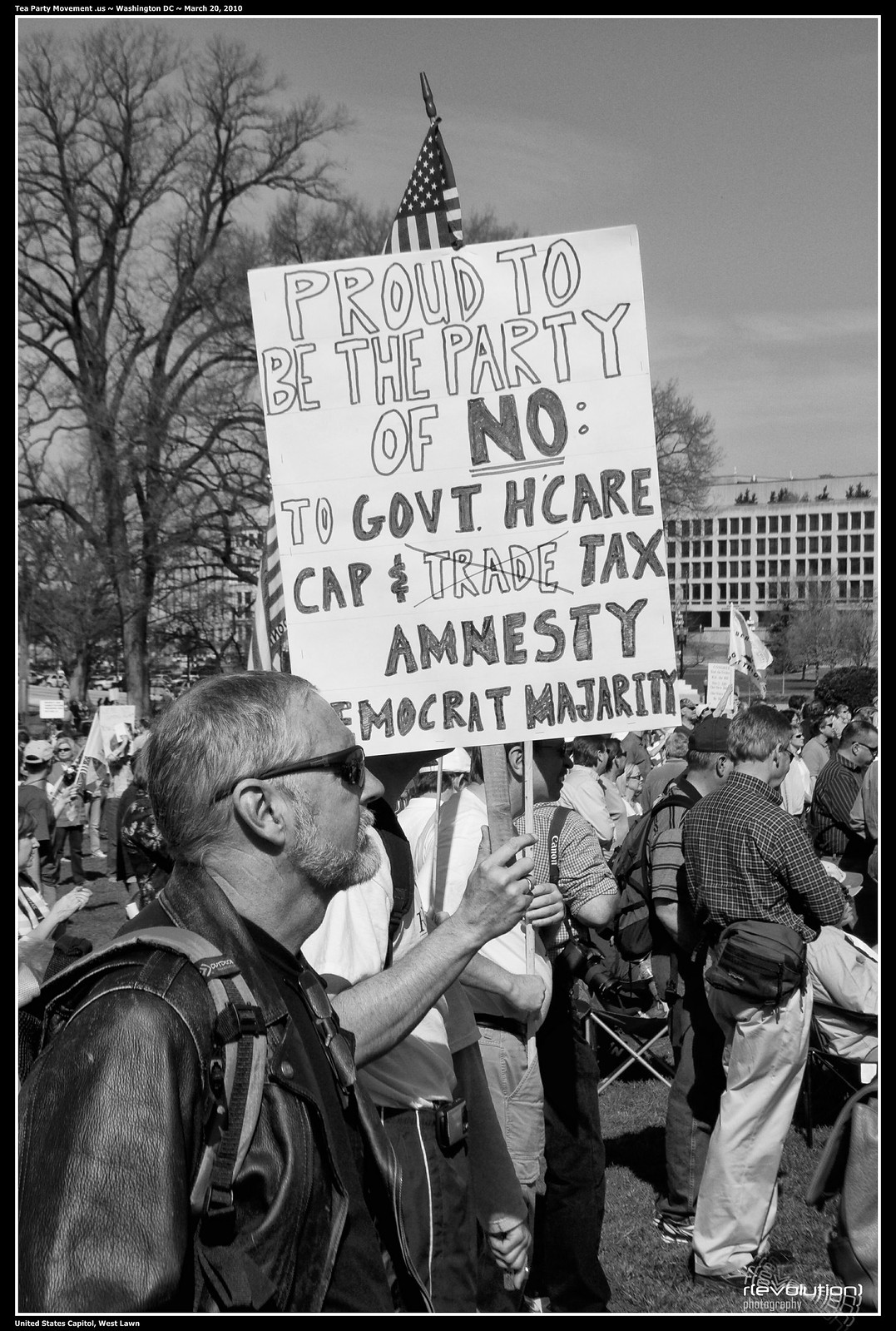In this black-and-white photograph taken outdoors, likely during fall or early spring, a large crowd has gathered in front of a building, possibly for a protest. In the foreground, on the bottom left, a man wearing a black leather jacket and a backpack stands prominently. He has a pair of sunglasses on and another pair hanging from his shirt around his neck. Right behind him, slightly to the right, a man holds up a handwritten white sign that reads, "Proud to be the Party of No" with specific objections listed: "No to Government Health Care, Cap and Trade (with 'trade' crossed out), Tax Amnesty, Democrat Majority." Some of these words are colored in, while others are outlined. Above the text on the sign is an American flag. The crowd extends into the background, where leafless trees and a building can be seen, emphasizing the season and the location of the gathering.